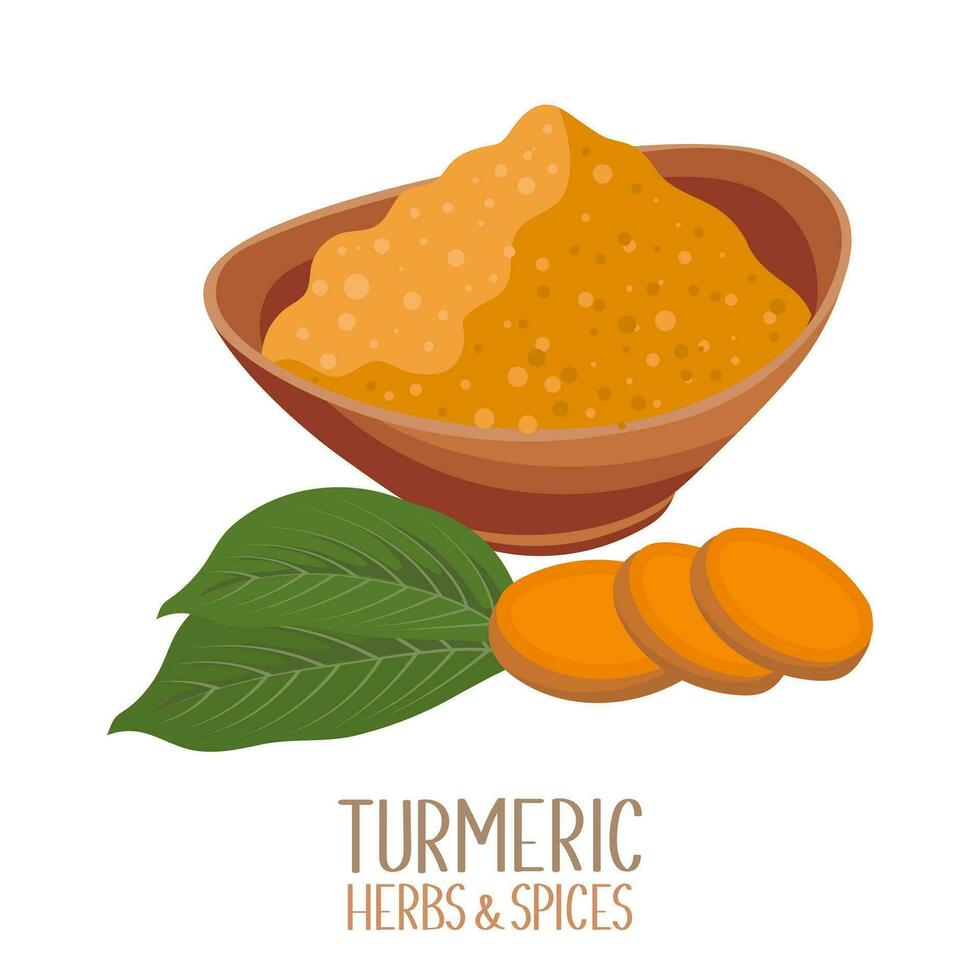The image is a minimalistic digital illustration set against a pristine white background, featuring elements related to turmeric. Prominently at the bottom, the text "TURMERIC, HERBS, AND SPICES" is written in varying shades of mustard and dark brown. Above the text, the illustration includes three round, orange turmeric slices arranged like fallen dominoes. To the left of these slices are two large, green leaves. At the top of the image sits a tall, clay-like bowl, depicted in various shades of brown. The bowl appears to be filled with turmeric powder, represented with a cream-colored base and a brownish tint, incorporating abstract squiggly lines and assorted tan dots to convey its granular texture. The overall artwork has a simple, cartoonish style, possibly designed as a branding image for a company’s product.